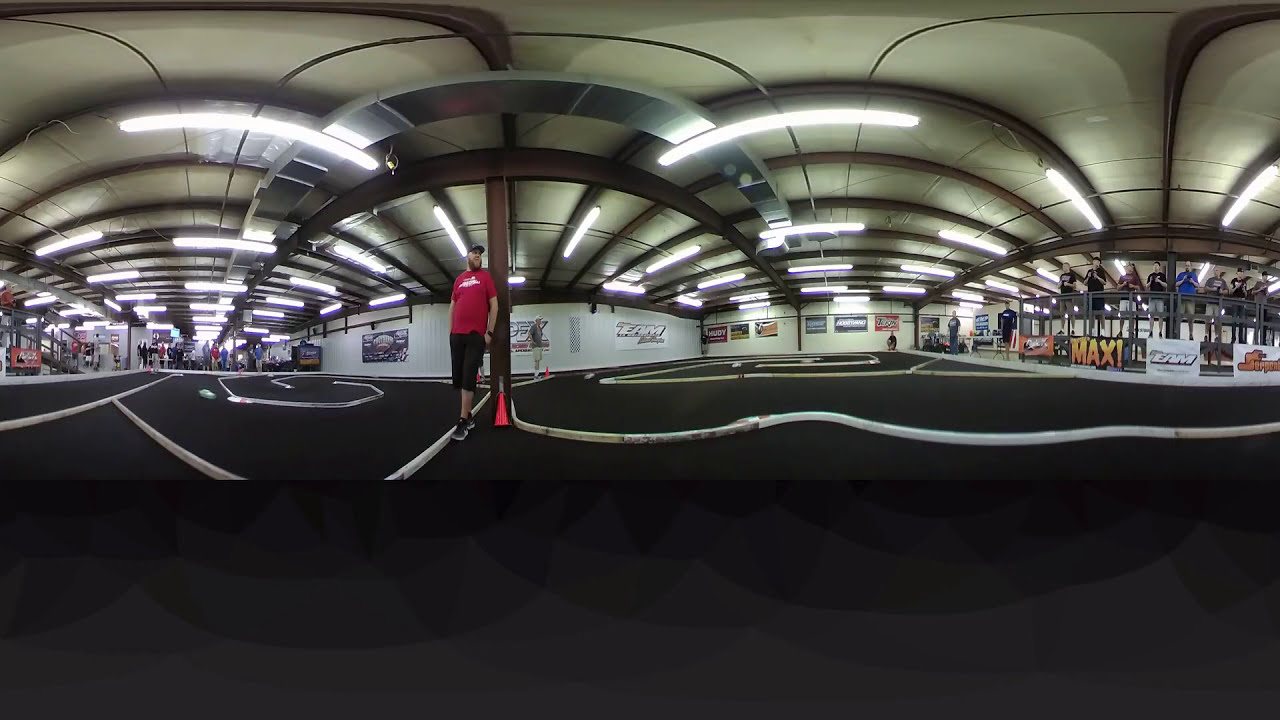This image captures an indoor sports arena, likely taken with a 360-degree camera, creating a curved and expansive view. Central to the scene is a man in a red shirt, black pants, tennis shoes, and a baseball hat, standing by a pole with a beard. The floor features white lines in various patterns, suggesting a track or sports field, and overhead fluorescent lighting illuminates the area. To the right of the man is a section with the patterned floor lines, and further right, there's a clothing store with a visible sign reading "Maxi" and mannequins on display. On the left side, an alleyway possibly leads to additional shops. The presence of people around and the spacious, open environment hints it could be an indoor gym or even an area designated for car racing, with spectators visible, perhaps waiting for an event. The scene is filled with a variety of colors including black, gray, white, red, blue, yellow, orange, pink, and purple.